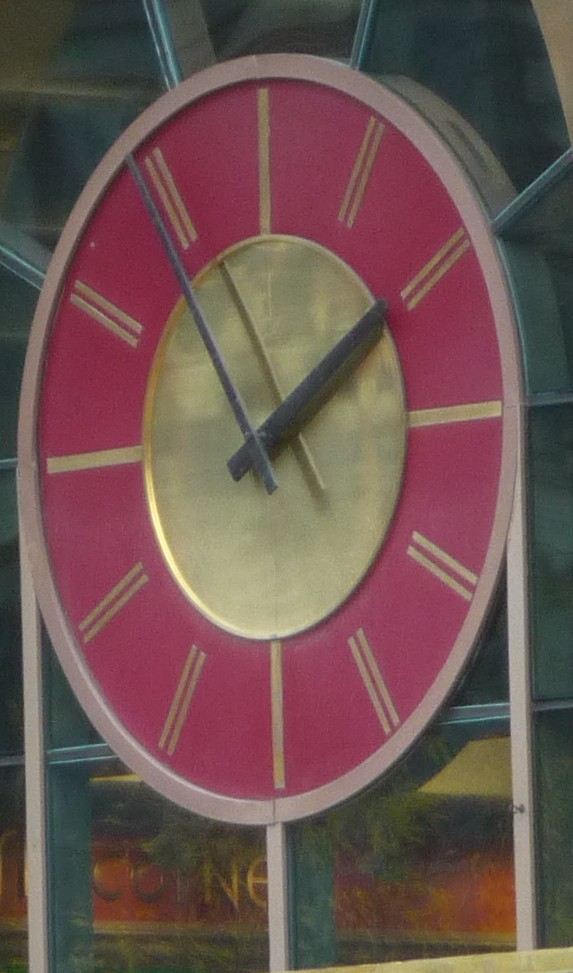The image depicts an angled view of a clock set into the front façade of a public shopping center, viewed from a slight diagonal perspective from the right-hand side. The clock has a circular design with a central golden circle and a surrounding red face. It features a minimalist style, marked only with golden lines instead of numbers or Roman numerals. The primary markers for 12, 3, 6, and 9 o'clock are single lines, while the other hour markers consist of double lines. The outer frame or bezel of the clock is pink, contrasting with its golden detailing. 

The clock hands, including the hour and minute hands, are black or dark gray and reflect off the golden central part of the clock face. The time displayed is five minutes to two. There are potential additional elements or reflections visible in the center, but their exact nature is indistinguishable.

This clock is integrated into a windowed structure that leads into a store. Through the clear glass beneath the clock, part of the store’s sign is visible. The sign is partially obscured by reflections and structural elements, but displays golden letters that seem to read "C O I N," possibly followed by another character partially hidden by the vertical strut framing the clock.